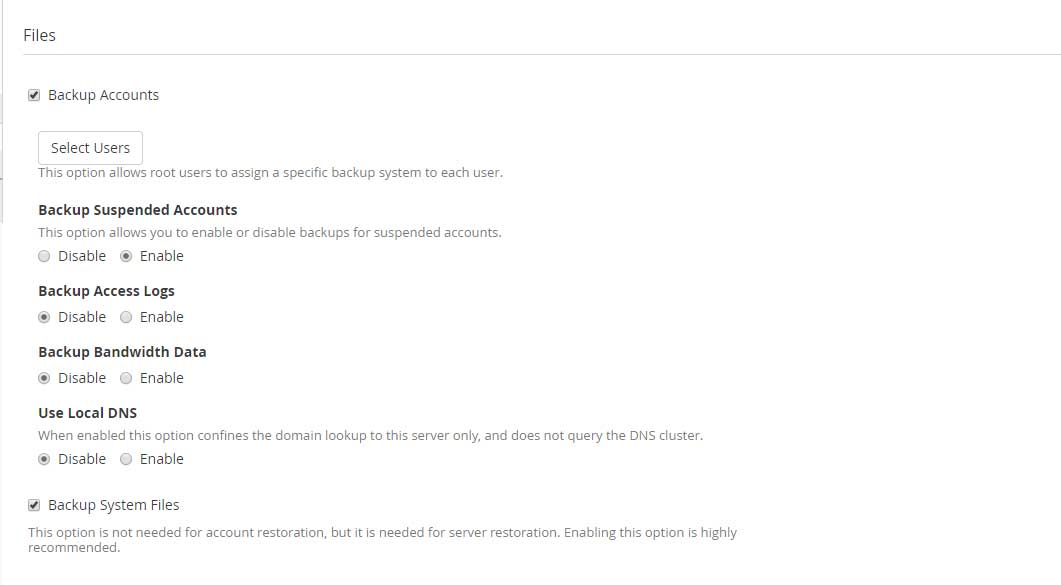### Detailed Caption:

This image showcases a settings interface for managing backup accounts on a computer system. At the top of the screen, a tab labeled "Files" is visible. Directly below, a section titled "Backup Accounts" is selected, highlighting its options for configuration. 

Within the "Backup Accounts" menu, the first sub-option is "Select Users," followed by a description: "This option allows root users to assign a specific backup system to each other." 

Further down, the menu includes an option for "Backup Suspended Accounts," which has toggle buttons for enabling or disabling the feature. 

The next option, labeled "Backup Access Logs," similarly provides toggle buttons to enable or disable the logging of backup activity. Following this, there is an option for "Backup Bandwidth" management.

The interface proceeds with an option for "Local DNS," followed by another section at the bottom titled "Backup System Files." Accompanying this option is an explanatory note: "This option is not needed for account restoration but it is needed for server restoration. Enabling this option is highly recommended."

Overall, this screen provides a comprehensive suite of settings for configuring various aspects of the backup system, ensuring that both user accounts and essential server files can be preserved and restored as needed.